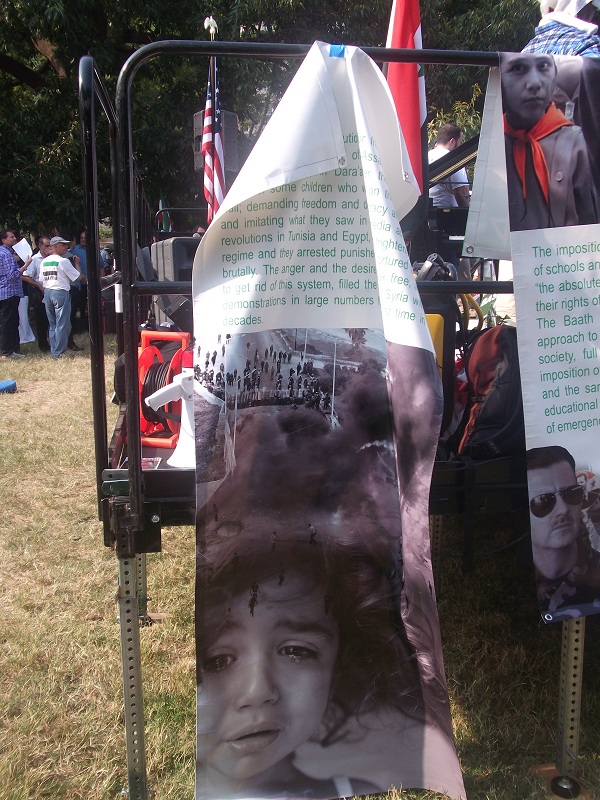The image depicts a bright, sunny day at an outdoor rally, featuring a portable stage adorned with various banners and flags. Central to the scene is a prominently displayed poster on the black railings of the stage, showing a heart-wrenching photograph of a crying child set against a chaotic, smoky background, suggesting an explosion in a war-torn area. Above the image, partially obscured text references revolutions in Tunisia and Egypt. Another banner to the right features images of a boy scout at the top and a man in sunglasses at the bottom. The stage, equipped with black adjustable legs, hosts speakers and electronic equipment, hinting at potential live music performances, reinforced by the presence of a piano. In the background, a crowd of people, some holding papers, and the presence of trees frame the scene. The American flag waves prominently in front, emphasizing the rally's location.